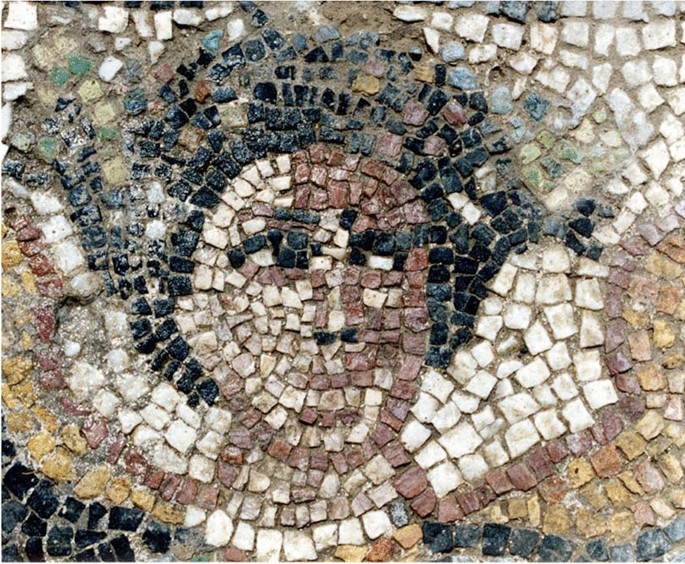This photograph captures a detailed and weathered mosaic embedded in a stone wall or brick-laid surface, depicting the visage of a person or figure with features reminiscent of an angel or an individual of African descent. The composition prominently features angular and somewhat irregularly shaped stones in varied colors, arranged with intricate care. The face is crafted primarily from a reddish layer for the skin, contrasted by a beige layer highlighting facial contours and white stones used for the eyes. The hair and eyebrows are defined using black stones, giving a textured, puffy appearance. 

Distinctive elements include a blue halo encircling the head, denoting an angelic aspect, while the wings are represented by a mix of white and rosy tiles bordered by reddish-brown stones. The neck's intricate gradient, shifting from dark brown to beige, further adds to the depth of the mosaic. The overall texture appears worn, reflective of ancient origins and exposure to the elements, adding historical intrigue.

The mosaic's surrounding area shows signs of decay, with stones displaced and patches of dirt and sand interspersed among the tiles. Adjacent to the figure’s hair, there are larger gaps filled with green and yellow stones amid sandy fragments, suggesting significant aging and possibly ancient Roman craftsmanship. This close-up image, captured in daylight, highlights both the enduring artistry and the inevitable passage of time evidenced by the mosaic's condition.